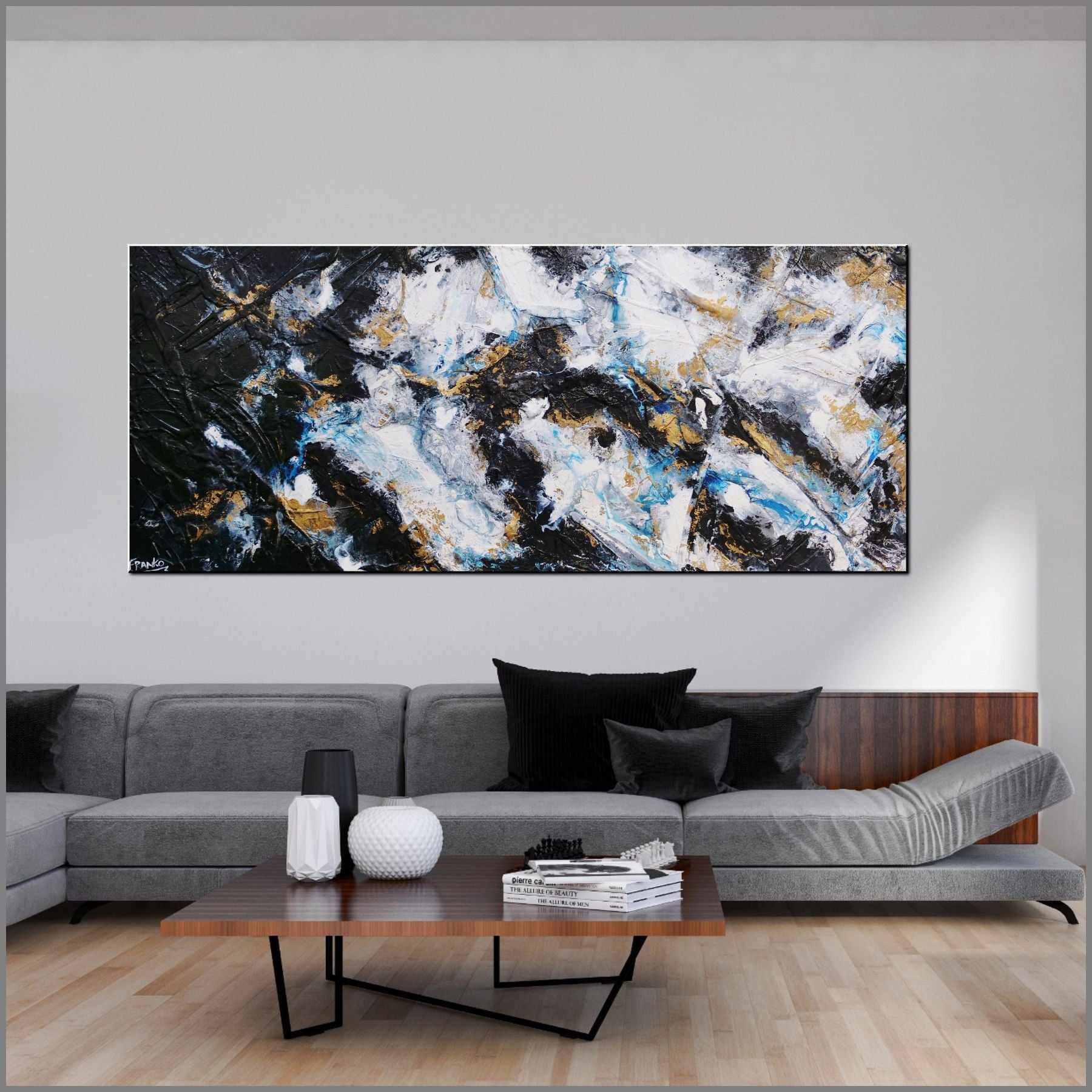This colour photograph showcases a stylish living room, possibly intended for a catalog or an online store. The feature wall in the background is a light grey shade, adorned with a large rectangular abstract painting characterized by swirling patterns of black, blue, beige, and white. The artist's signature, "F-P-A-N-K-O", is visible in the bottom left-hand corner of the painting.

Dominating the room is a modern, sleek gray sectional couch, positioned at an angle that suggests it extends beyond the photo's left edge. The couch features black cushions, with one cushion on the right side notably angled upwards, hinting at a recliner or convertible bed mechanism. A segment of the couch's backrest reveals dark wooden paneling with striped detailing, adding a touch of sophistication to the piece.

In front of the couch sits a square wooden coffee table with unique black iron legs shaped asymmetrically, providing an artistic element to the room. The table is adorned with a trio of vases—two white and one black—and a neat stack of white books or magazines. The floor beneath these furnishings is a light brown wood with beige paneling, adding warmth to the room's modern aesthetic.